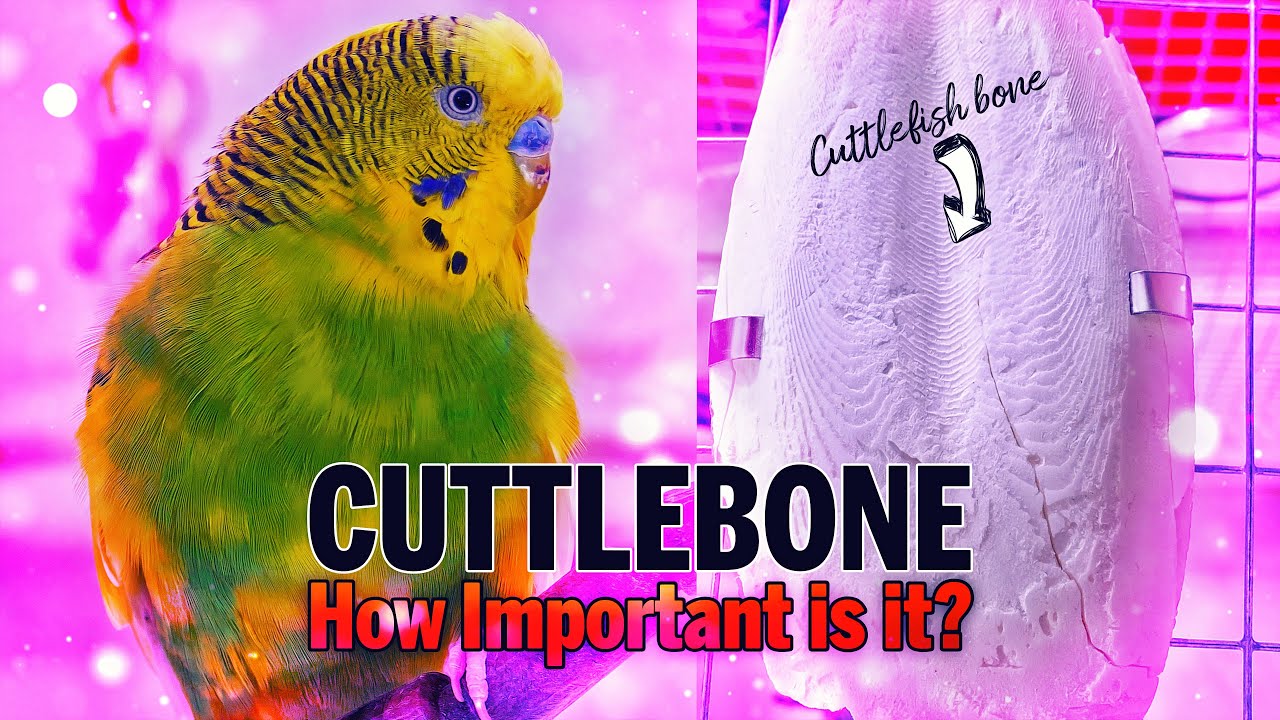The image is a vibrant and detailed poster divided into two sections. On the left side, there is a close-up of a small parrot-like bird with predominantly yellow feathers, green on its sides, and black on the back of its neck. The bird features distinctive blue-purple rings around its black eyes and its blue beak nestles closely to its chest. It sits against a mainly purple background adorned with subtle white spots.

To the right, the image displays a large, white cuttlebone hanging downwards, highlighted by a curved white arrow pointing toward it. The cuttlebone bears the text "Cuttlefish Bone" in black cursive, drawing attention to its importance. Behind this, the background mirrors the left side’s color scheme with an additional overlay of purple lines and a grid pattern in the upper right corner, featuring purple edges and orange squares.

At the bottom of the poster, written in a combination of black and red text, the caption asks, "Cuttlebone, how important is it?" indicating a focus on the nutritional value of the cuttlebone for the bird's health.